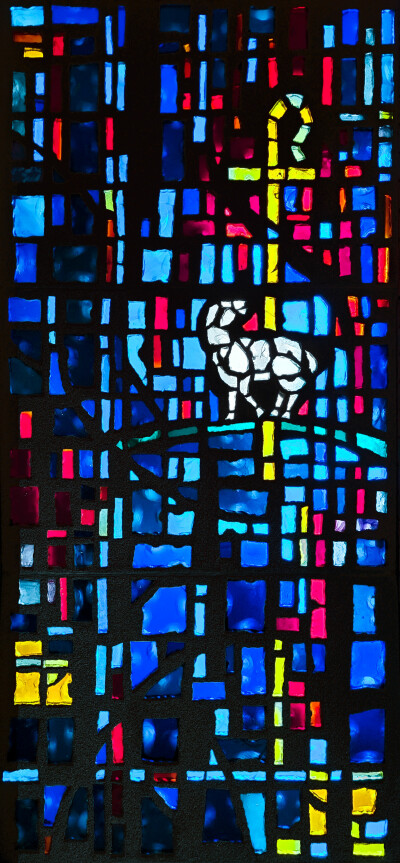This photograph captures a stunning stained-glass window, likely from a church, set against a plain white background. The window itself is rectangular and vertically oriented, with the majority of its colored glass pieces showcasing different shades of blue, including dark and light hues. The image prominently features a small white lamb that seems to be sitting on a light blue hill in the center towards the top of the window. Behind the lamb, a yellow shepherd's cross with some blue detailing on its curved handle ascends diagonally towards the upper right corner. Additional colors in the stained glass include red, green, and pink, all neatly segmented by black lines. The intricate design consists of many small, square-ish glass pieces making up this detailed and vibrant window. The photograph seems to be taken at night, as there is minimal light streaming through the window, highlighting the vivid colors and patterns captured within the stained glass.